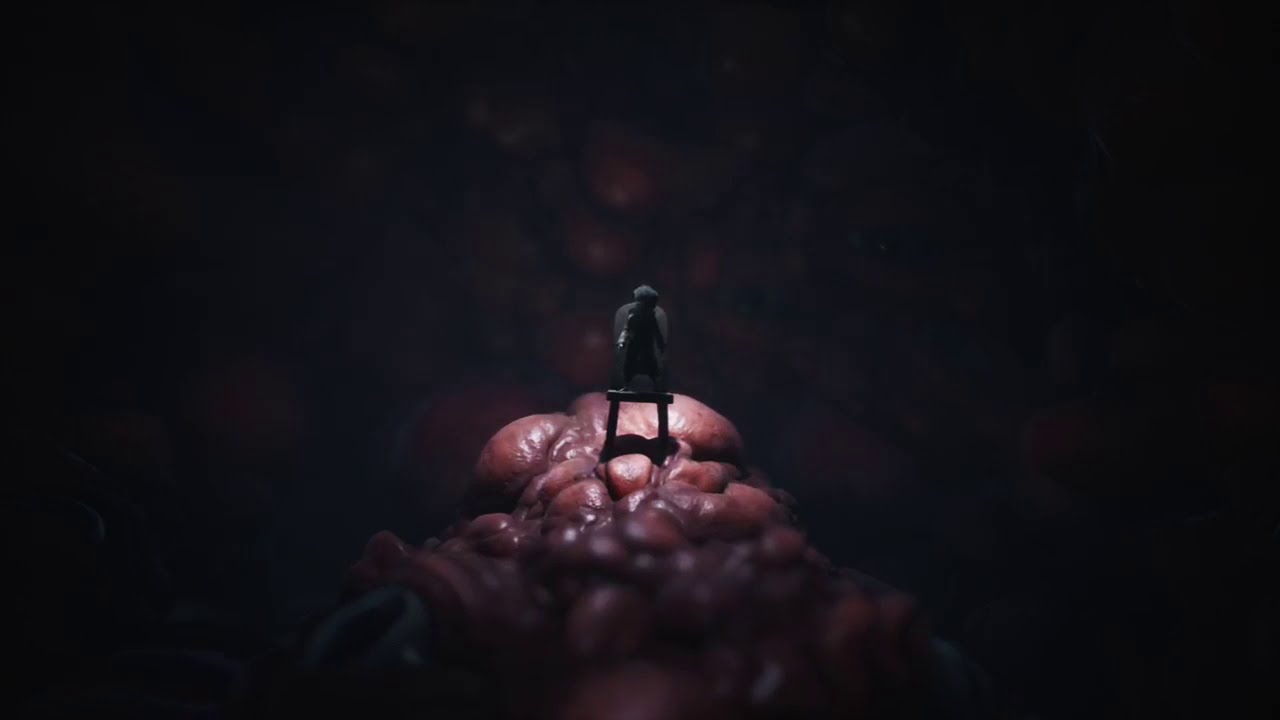In the image, there is a heavily darkened background featuring bumpy, reddish-pink, flesh-like material, reminiscent of the inside of an organ or an alien's skin. This lumpy texture extends throughout the scene, creating a surreal, slimy appearance. At the center of the image, atop a black wooden chair, stands a completely dark, shadowy figure with stark white sleeves. The chair appears precariously balanced on a mountain of this brainy material. In the lower corners of the image, pairs of white, oval-shaped eyes gaze out from the organic mass. An additional eerie eye looms faintly in the right background, watching the figure. The overall effect gives the impression of a fantastical or video game-inspired scene, where the figure might be standing on the nose of a massive, obscured creature.